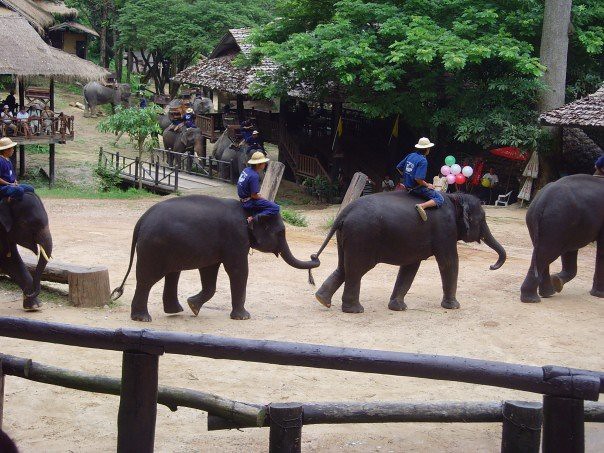In this image set in an outdoor elephants sanctuary, likely in Thailand, four elephants are walking from left to right in a line, seen from varying angles. The elephant on the far left is partially visible, displaying just its face and a leg, while the next two elephants show their full side profiles. The elephant on the far right reveals only its back end and three legs. All four elephants are clearly in motion, each with at least one leg raised.

There are three people riding the elephants: one on the far left elephant, and two in the middle. The middle elephants feature riders clad in blue jeans, royal blue shirts with white insignias on the back, and white safari-style hats. It is not clear if there is a rider on the elephant on the far right. 

The elephants in the center exhibit additional interaction; one has its trunk wrapped around the tail of the one in front. These elephants are a gray color, contrasted against the earthy dirt path they tread. The scene’s ambiance is enriched by a wooden fence in the foreground and lush greenery, including trees, in the backdrop.

Multiple colorful balloons are dispersed throughout the scene. The setting also contains several structures, possibly pavilions with tourists observing the elephants. In the background, more elephants are present, some of which are carrying additional riders.

A large hut with a thatched roof, connecting bridges with bamboo railings, and a stand with balloons enhance the lively backdrop. The elephants and their riders appear in an environment that could be on the edge of a rainforest, portraying a vibrant and active sanctuary scene.